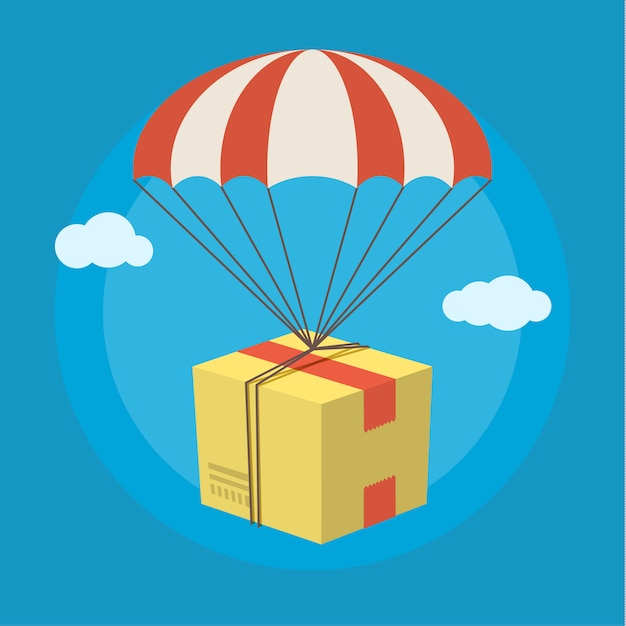The image is a detailed graphic illustration of a yellow package being gently lowered by a parachute. The package is wrapped with two pieces of red tape that have scraggly edges, indicating they weren't cut perfectly straight. The parachute resembles an umbrella, featuring vertical red and green stripes, and is connected to the package by multiple strings. The entire scene is set against a turquoise background that forms a square shape. Concentric blue circles radiate outward from the center, transitioning from a light turquoise in the middle to progressively darker shades of blue. Adding to the sky-like atmosphere, there are two small clouds positioned on either side of the package, contributing to the sense of it floating down safely.